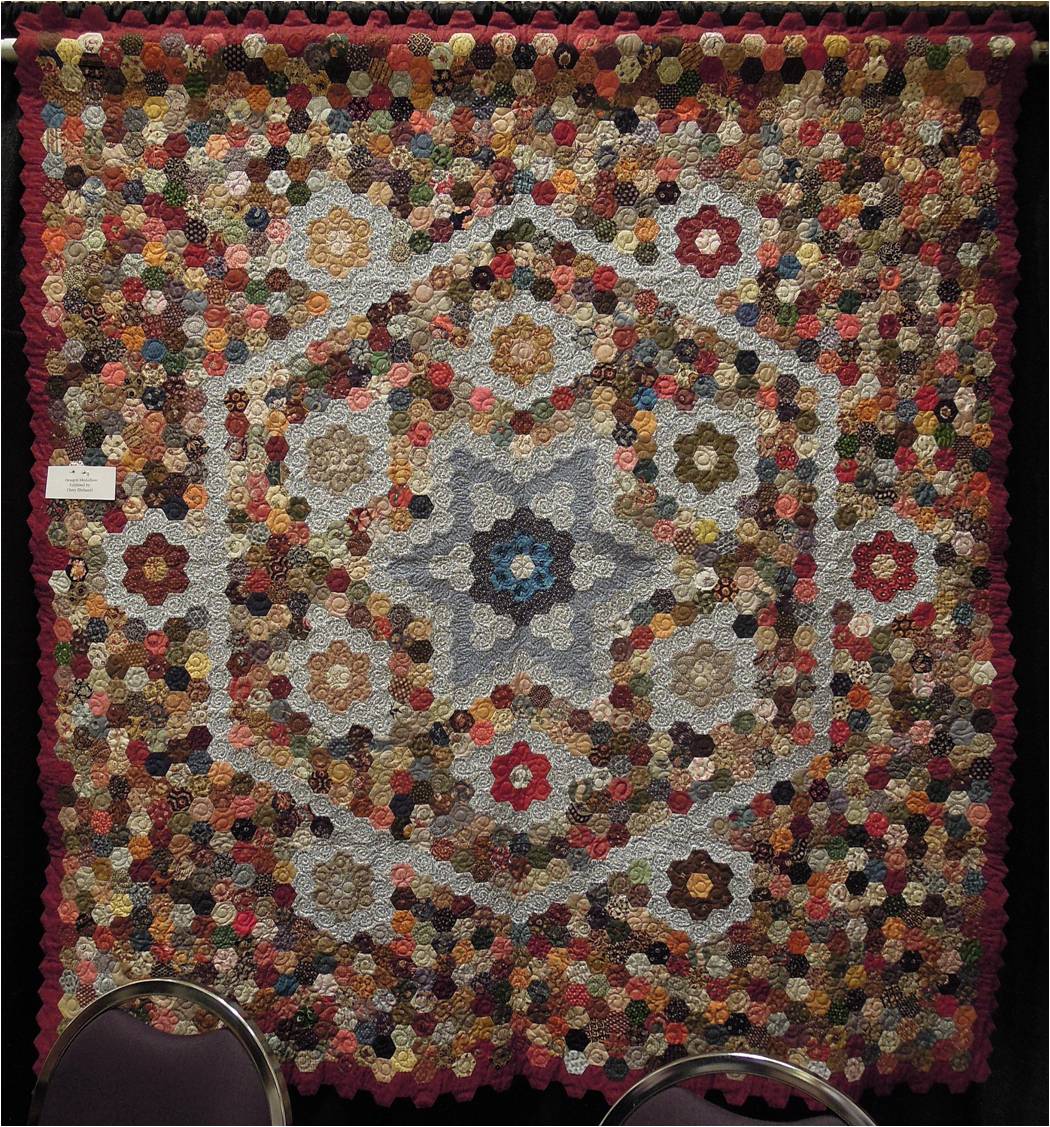This is a photograph of a detailed and colorful hexagon quilt, displayed prominently on a black wall. The quilt hangs from a white-painted rod, mounted like a curtain rod. It features a burgundy red border, with numerous small, hexagon-shaped fabric pieces of various colors and patterns meticulously sewn together. These hexagons come together to form a central star, surrounded by six flowers, each bordered by another hexagonal pattern.

Each flat side of the hexagonal border around the central star and flowers showcases a flower of a different color: tan, brown, red, dark red, yellow, and reddish-brown. In the heart of the star, there's one large flower in shades of white, gray, and blue. This quilt is complemented by the presence of two silver-framed chairs with brown backs placed in front of it, enhancing the room's cozy ambiance.

Additionally, there may be an informational piece or a sale price sign placed near the quilt, suggesting that it could be displayed in a venue where such handcrafted items are sold. Despite the somewhat dim lighting, the quilt's rich array of colors stands out, making it a perfect piece for a fall setting.